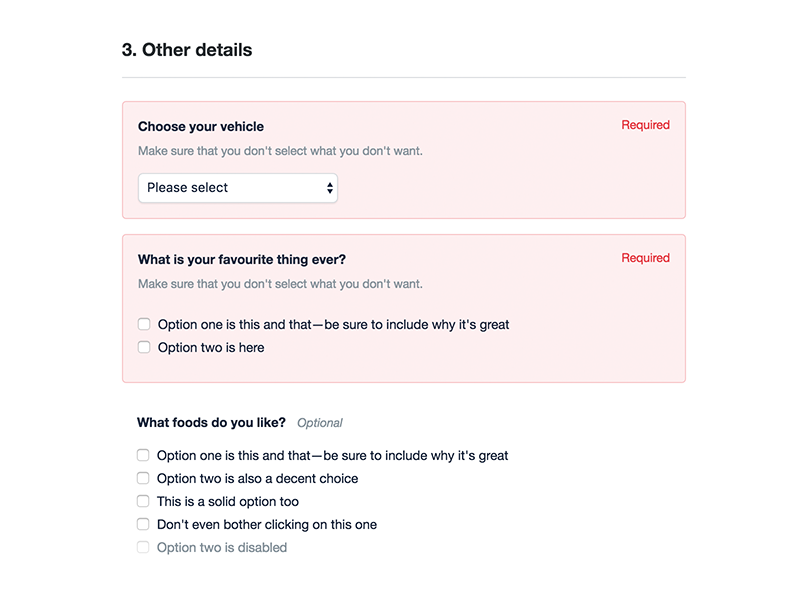This image captures a computer screen displaying an online form. At the very top of the screen, the numeral "3" is prominently visible, followed by the text "other details." Below this heading runs a faint, skinny gray line that stretches horizontally from the left to the right side of the image.

Underneath this line are two noticeable pinkish rectangles. In the upper right corner of both rectangles, the word "Required" is highlighted in red print.

In the first rectangle, on the top left, the black print reads "Choose your vehicle." Directly beneath this, written in gray print, is a reminder: "Make sure that you don't select what you don't want." Following this instruction is a dropdown box labeled "Please select" in black print, accompanied by an up-and-down arrow indicating a selection option.

The second rectangle features a heading in black print that states "What is your favourite thing ever," notably spelling "favourite" with a British "u." Below this, in gray print, is the same reminder as before: "Make sure that you don't select what you don't want." The form then presents two options available for selection.

Towards the bottom of the screen, there's a section titled "What foods do you like." This part of the form is marked as optional. It offers five checkboxes for the user to select their preferred food options.